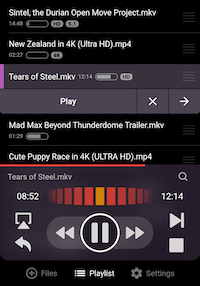The image displays a media player interface with various playback options, such as play and pause buttons, indicating its ability to handle audio-visual content. The interface exemplifies compatibility with different file formats including MP4 and MKV.

At the top section of the interface, there is text that reads "Sintel, the Duran, OpenMoveProject.mkv," alongside a timestamp of "14:14/48:00," indicating the elapsed and total duration of the video. Adjacent to this, there are icons representing the status, HD (High Definition), and 5.1 surround sound capabilities.

Further down, another media entry is visible, titled "New Zealand in 4K (Ultra HD).mp4," with a duration of "2:27." This entry prominently features a 4K symbol, underscoring its high-resolution quality.

Near the bottom of the interface, a third entry titled "Tears of Steel.mkv" is displayed with a runtime of "12:14." The consistent use of file formats (MKV and MP4) and detailed metadata, such as duration and resolution, provide a comprehensive overview of the available media content.